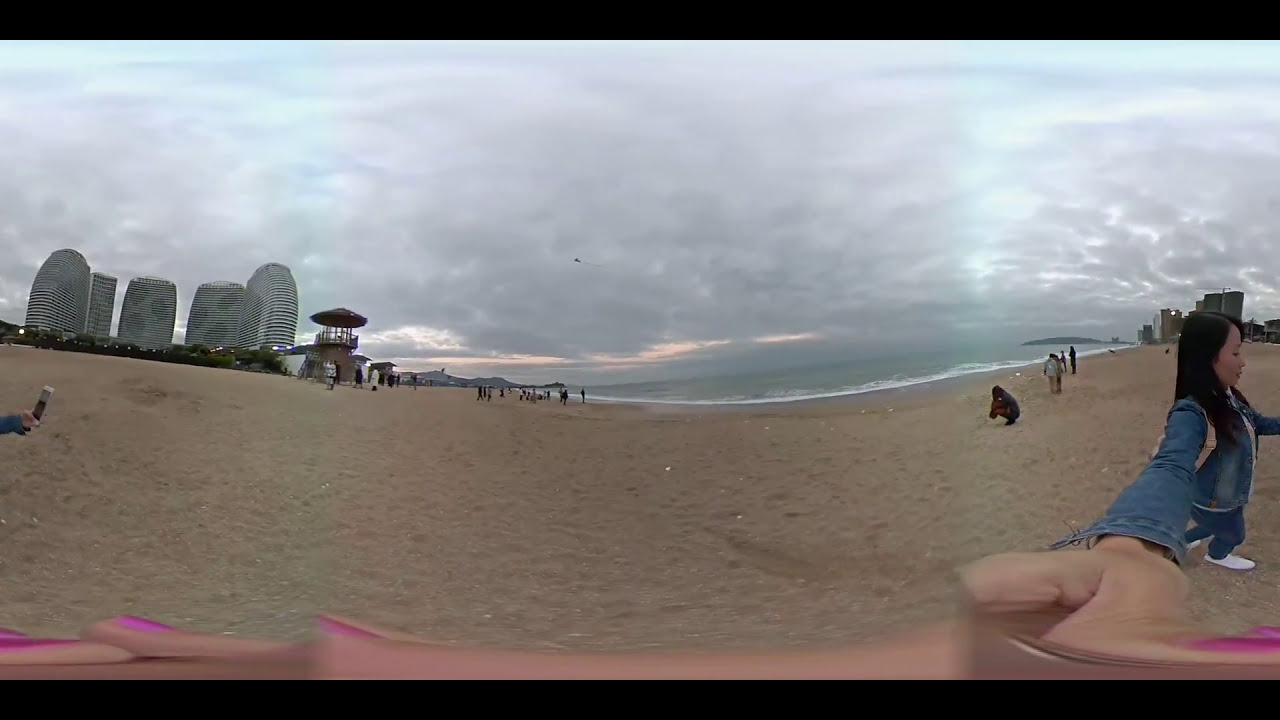In this wide-angle photographic image, we're presented with a dynamic and somewhat curved beach scene. The landscape is dominated by a mixture of elements: a vast, tranquil ocean with gentle waves washing onto the sandy shore, and a sky heavily laden with dark, black overcast clouds, though patches of blue and sunlight peek through. 

In the background, to the left, a series of beehive-shaped stone structures stand, adding an intriguing architectural element that contrasts with the natural surroundings. These structures don't resemble typical buildings, suggesting they might be artistic installations or ancient constructions. Adjacent to these structures is an elevated gazebo with a gabled roof and banisters. Behind it, individuals stand, including a man attired in a long, white, Middle Eastern or Indian-style shirt paired with black pants.

The foreground features a woman in profile, wearing black pants, a blue denim jacket, white sneakers, and sporting pink fingernails. She appears to be attempting a selfie, her hand prominently distorted by the camera's wide angle. Her dark hair and Asian appearance are subtle details that personalize the scene. On the same sandy stretch, another woman kneels or squats, gazing at the ocean, while more people dot the beach, looking outward, suggesting a contemplative atmosphere possibly influenced by the cooler weather implied by their jackets.

On both the left and right sides of the image, tall buildings—likely hotels or resorts—border the beach. These structures lend a backdrop of urbanization to the otherwise natural and serene setting. 

Overall, the image captures a complex, multi-layered scene juxtaposing natural beauty, human presence, and curious architecture under a dramatic, cloud-filled sky.